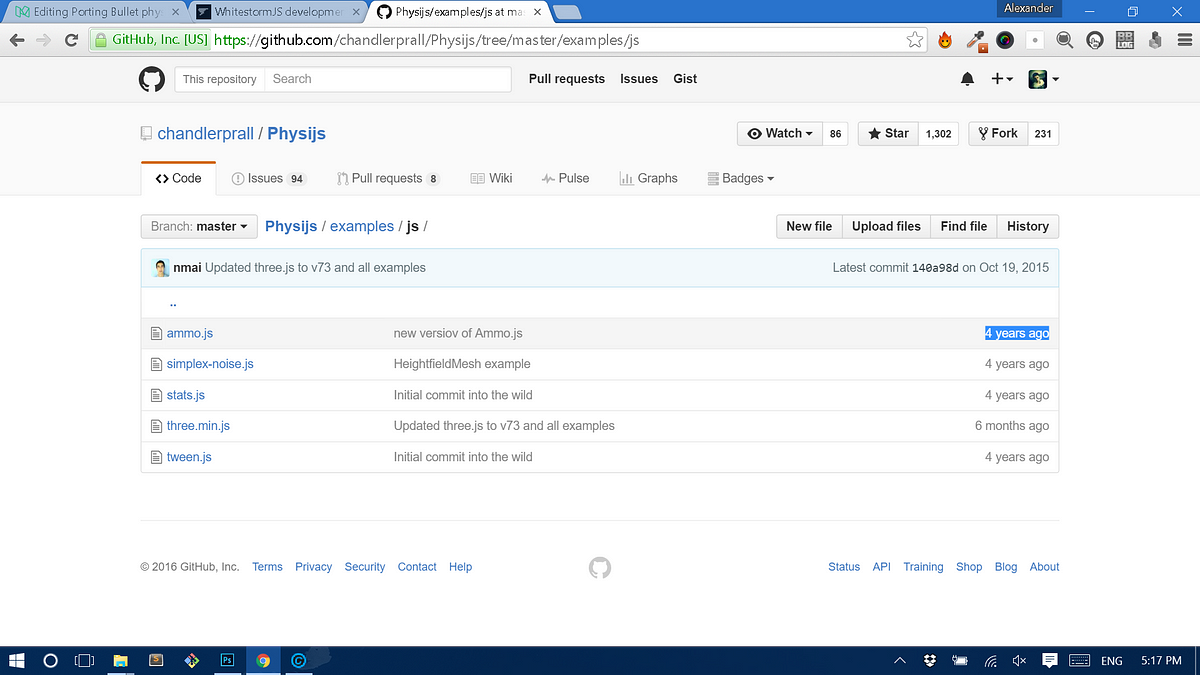This image captures a screenshot of the GitHub website, specifically displaying a repository page. The browser tab shows GitHub's URL (github.com) and there are two additional browser tabs open next to it. The main GitHub tab is currently active. The screenshot highlights a repository that has recently been updated, marked by the text "Updated V73 and all examples." Below this update, there is a list of five clickable links, each accompanied by an icon on the left. The links appear to relate to different versions or components, as indicated by their names. Moving to the right side of each link, there are descriptions, such as a "new version of Ammo." Further to the right, time markers indicate the age of these updates; four of them are labeled as updated four years ago, while one shows an update from six months ago.